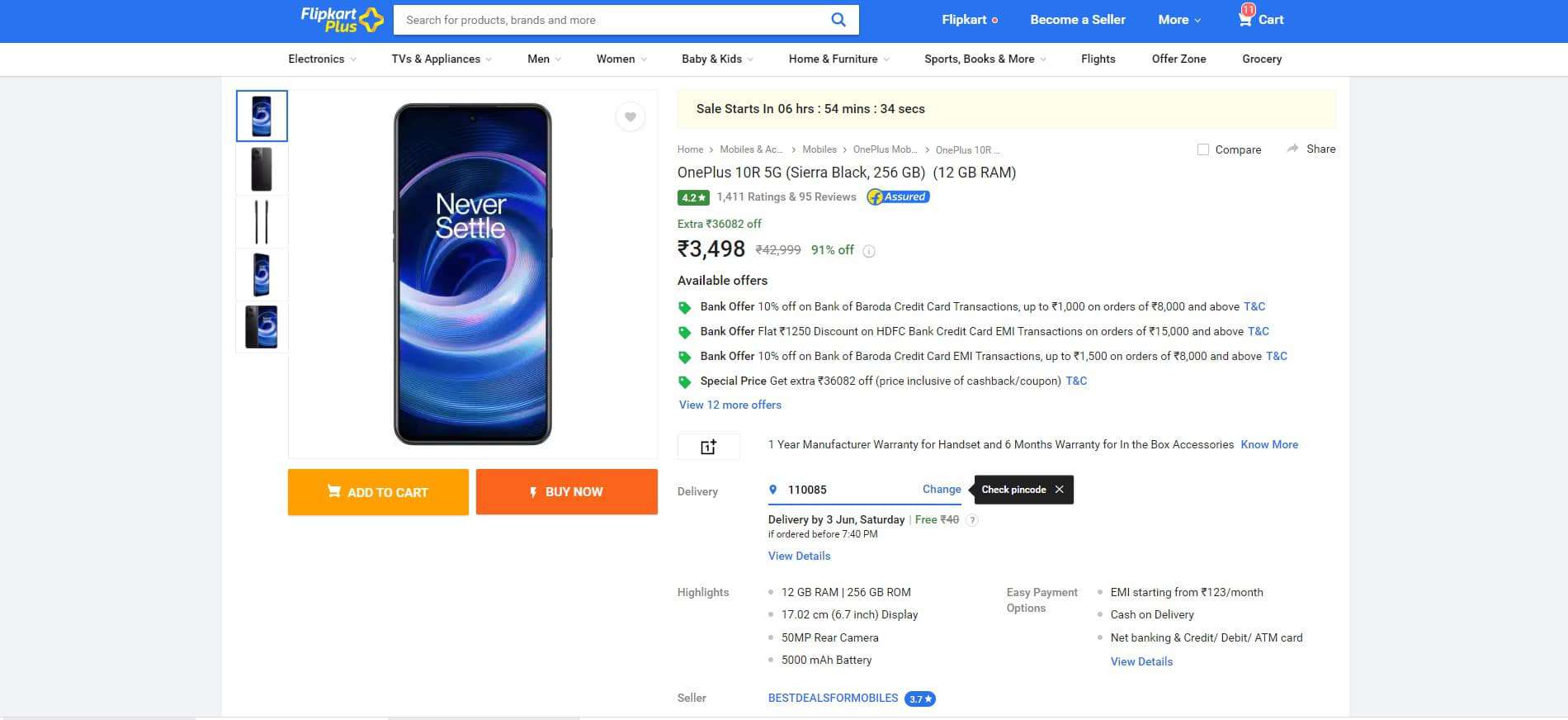This webpage, sourced from Flipkart, appears to display a listing for a mobile device. The device in question is the OnePlus 10R 5G, indicated below the price, which is listed in pounds, suggesting it is tailored for an English-speaking market. The webpage design and layout suggest a peer-to-peer selling platform rather than a direct-from-manufacturer site. Despite the OnePlus name implying otherwise, the design of the mobile device closely resembles that of an Apple iPhone, raising ambiguity about its brand. It is unclear from the listing whether the product is a brand-new item or a refurbished device being sold by a reseller.